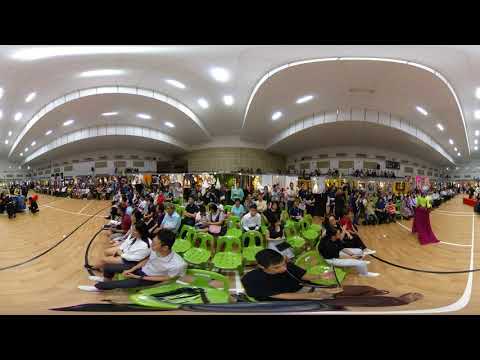The image depicts an indoor gathering set in a gymnasium or auditorium with unique architectural features. A large crowd of people, some standing but mostly seated in bright lime-green plastic chairs, are scattered across the brownish wooden gymnasium floor marked with various white and black stripes, typically used for sports courts. The backdrop includes distinctive architecture with a white, beveled ceiling illuminated by lights, which reflect brightly across the surface. White walls surround the space, and the center features a giant yellowish-brown pillar between the walls. The scene appears slightly distorted, as though taken through a specialized lens. Despite the distance blurring individual details, a central man in a black shirt and two individuals in white shirts nearby are discernible amidst the bustling crowd, suggesting an organized event or fair.